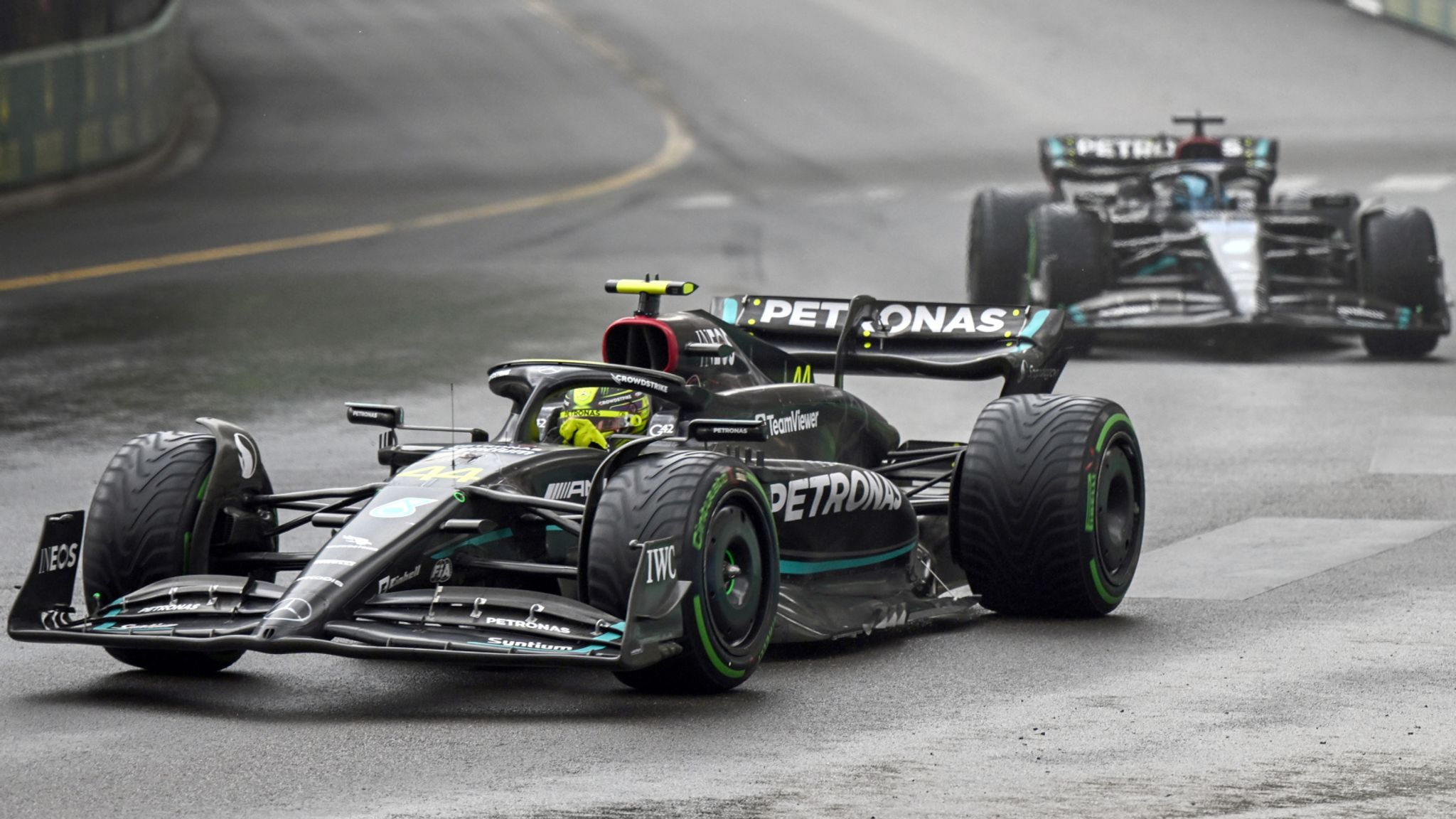This image showcases two sleek Formula One race cars navigating a left curve on a concrete racetrack. Both cars, predominantly black, belong to the same team and feature identical sponsorship liveries. The large white text "Petronas" is prominently displayed on the rear spoilers and the right sides of the cars. The leading car, identifiable by the number 44 and a visible Mercedes logo on its front tip, has additional sponsor logos such as IWC and Team Viewer. The driver of the front car sports a neon green helmet and matching gloves, contrasting with the vibrant blue helmet seen in the following car. Both vehicles are equipped with sizeable, thick black tires, marked with striking green stripes on the sidewalls, adding to their aggressive, low-to-the-ground, and aerodynamic design.